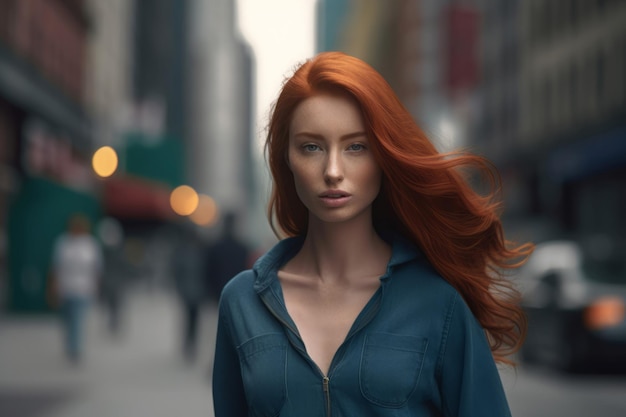This digitally enhanced photograph captures a fair-skinned, young red-haired woman, appearing to be in her 20s, as she walks down a bustling city street. Her striking red hair, parted on her left, cascades in loose waves past her shoulders. She has blue eyes, red eyebrows, a thin and graceful nose, and slightly open pink lips, revealing a glimpse of her teeth, though her expression is neutral.

Her attire consists of a blue collared top—possibly a jean or button-down shirt—unzipped and open at the V-neck, revealing a bit of cleavage and her collarbone. She stands out vividly against the very blurry backdrop, which suggests a lively urban setting, reminiscent of a place like New York City. In the out-of-focus background, one can discern tall buildings, people moving on the sidewalk, cars, and illuminated street lights. The composition implies her confident stride, as if she is focused or determined, heading towards the camera and capturing the viewer's attention amidst the city's hustle and bustle.